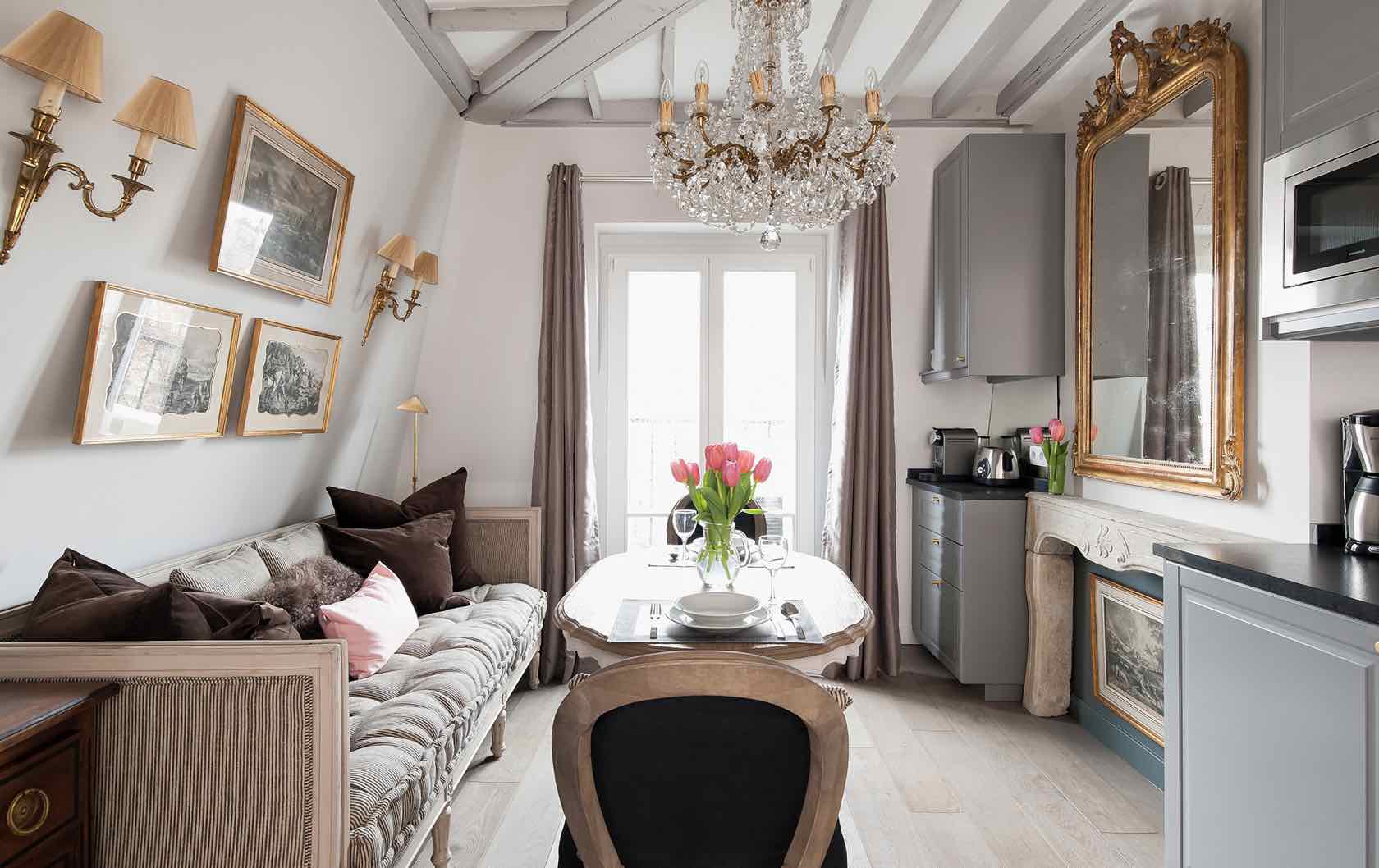This photograph captures the inside of a cozy, multi-functional room on the upper floor of a house, identifiable by the tapered ceiling design. The room is illuminated by natural light streaming through a large window or possibly a door, adding to its airy ambiance. The ceiling features white wooden beams and a central chandelier that adds a touch of elegance. The walls are painted in a blend of white and light pink, with the predominant color being white.

On the right side of the room, a large golden-framed mirror hangs above a functional space that combines a countertop, potentially gray in color, and a kitchenette equipped with essentials like a microwave, kettle, teapot, and toaster. Beneath the mirror is a space adorned with a painting, styled where one might expect a fireplace. The lower right corner also features a small gray cabinet with a matching darker gray countertop.

The left side of the room includes a beige couch with wooden accents and a pink pillow, offering a cozy seating arrangement. Adjacent to the couch is a brown end table, adding warmth to the decor. Three framed pictures with white backgrounds and gray designs are mounted on the wall, while two hanging lights in the far left corner provide additional illumination. The center of the room features a table set with wine glasses and a tucked-in chair, indicating a dining or lounging area. Overall, this inviting space seamlessly blends elements of a living area, kitchenette, and dining nook.